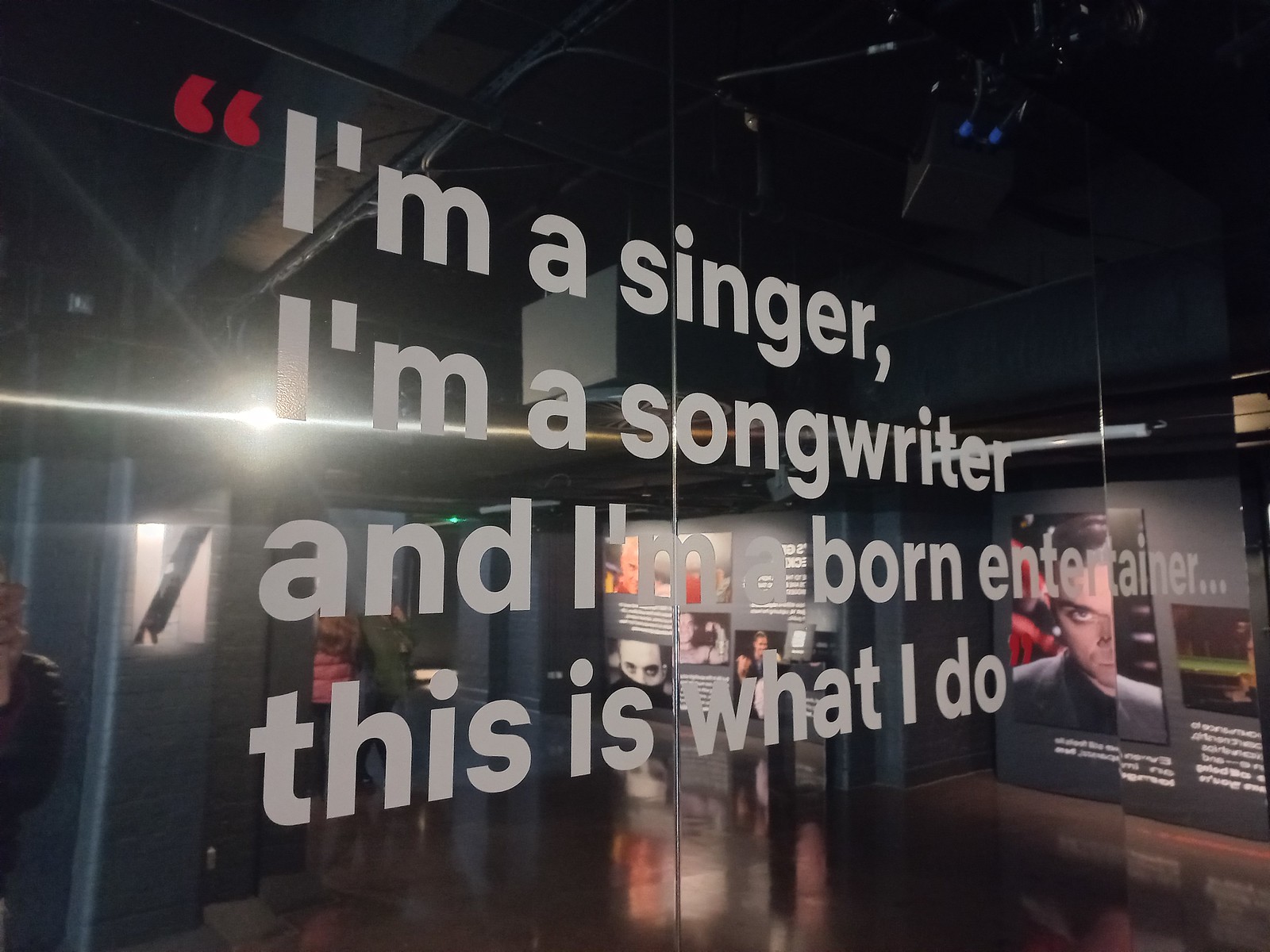The image depicts a notable quote displayed on a glass panel, likely situated within a museum. The central text reads, "I'm a singer, I'm a songwriter, and I'm a born entertainer. This is what I do." The lettering is prominently white, with vibrant red quotation marks, contributing to an engaging visual presentation. The backdrop features predominantly black walls and a dark gray floor, enhancing the text's clarity and impact. Surrounding the glass panel are additional entertainment artifacts and images of artists, suggesting an exhibition devoted to the entertainment industry. Observers might notice mirrors and reflective surfaces in the vicinity, indicating a thoughtfully arranged space to enhance the viewing experience. The quote and the artifacts create a compelling focal point, inviting museum-goers to pause and reflect on the rich legacy of performers and entertainers.